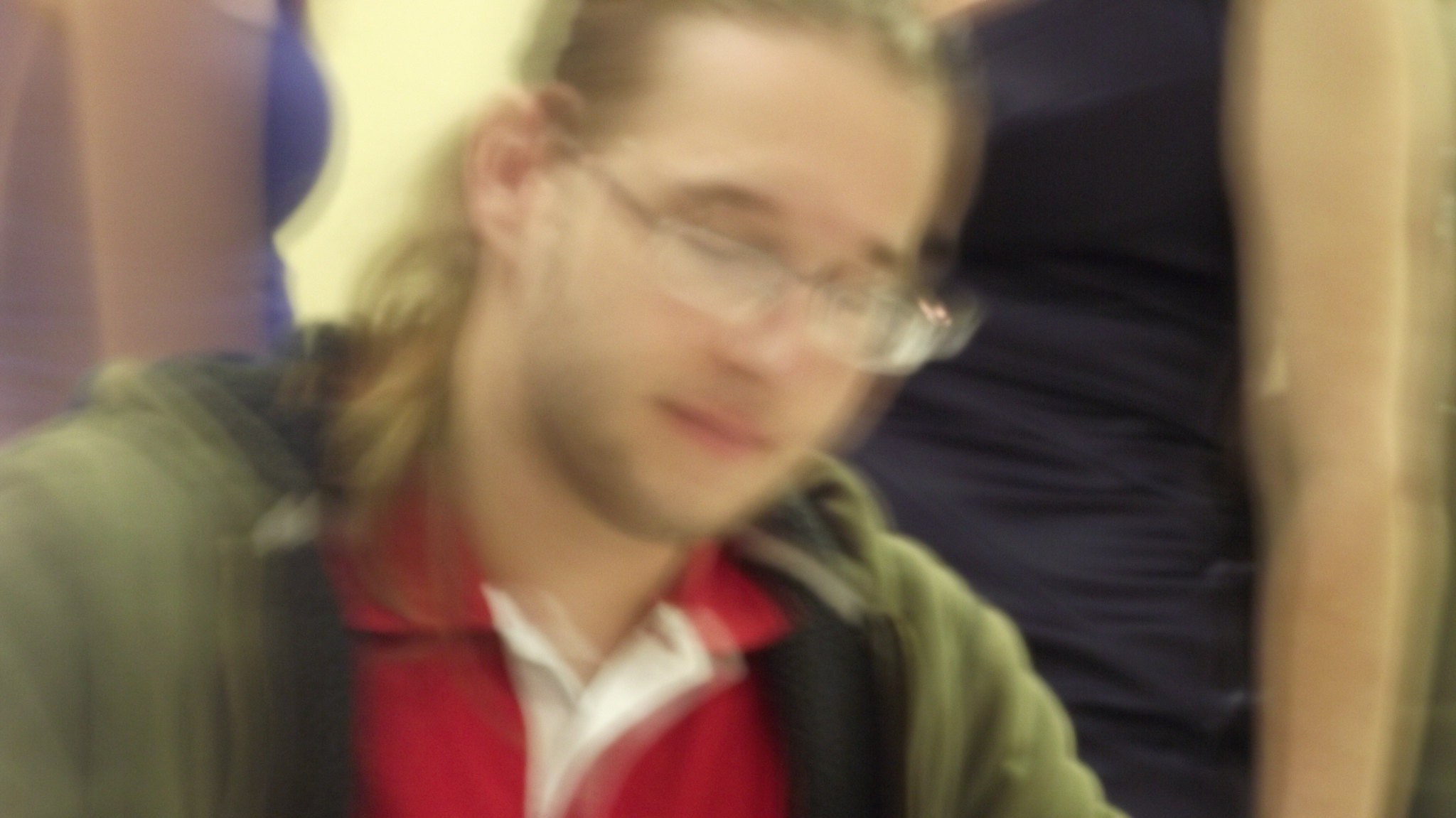The image is a very blurry capture, likely taken in motion, featuring a young white man with fair skin. His long, tied-back blonde hair and stubbled beard are particularly notable. He wears rectangular, clear-lensed glasses with brown or black frames, and his eyes appear closed as if blinking due to the motion blur. His attire includes a green khaki-colored hoodie over a red shirt with a white-striped collar. Straps, possibly from a backpack, are visible across his shoulders. In the background, two additional figures can be discerned; both appear to be women wearing sleeveless dresses, one black and the other purplish. One woman's blue shirt is also partially visible in the frame. Despite the presence of these background figures, the overall image remains indistinct due to its significant blurriness.